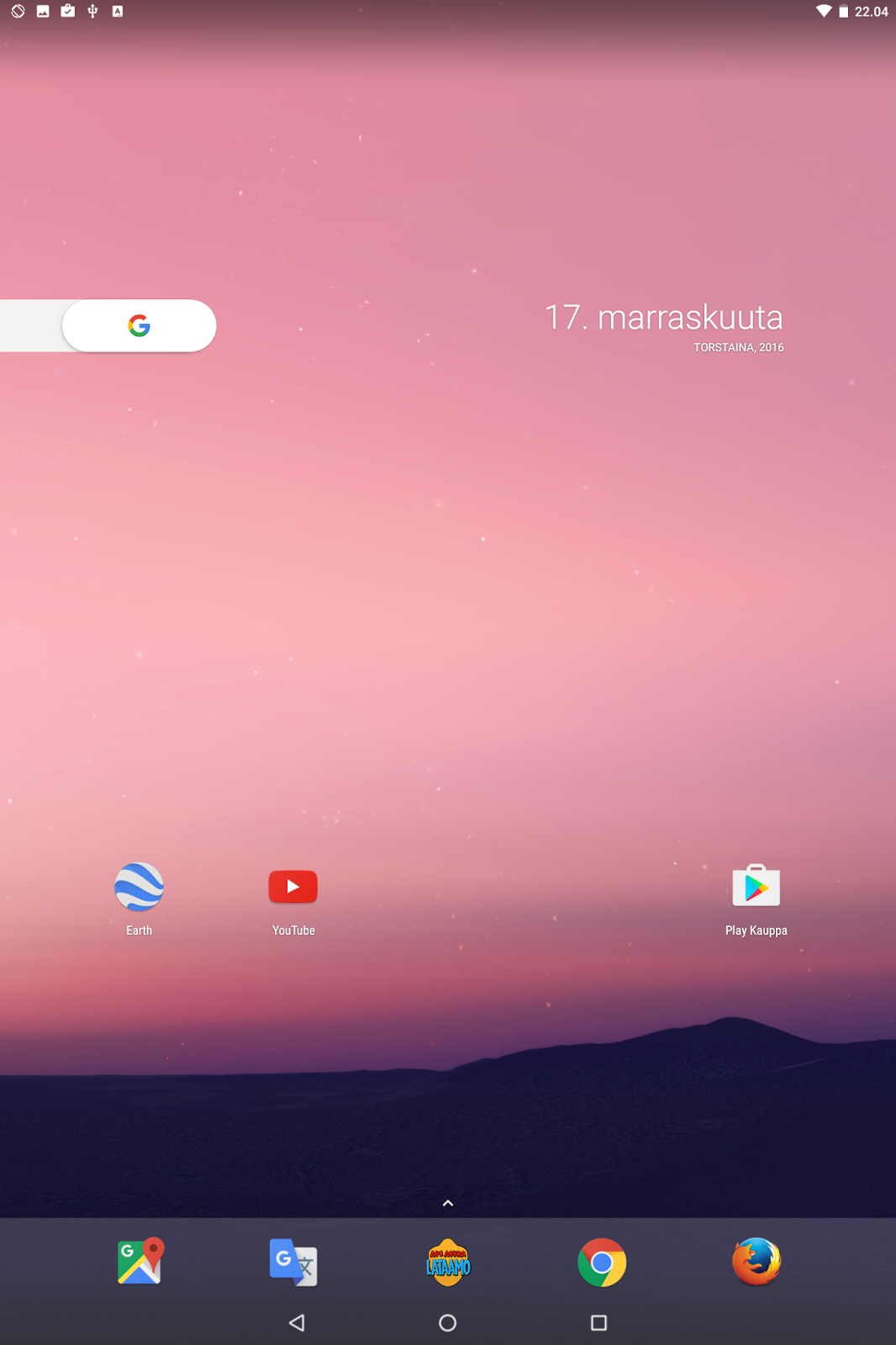This image is a detailed screenshot of an Android tablet's home screen. The background captures a gradient that transitions from pink to purple, evoking a serene atmosphere reminiscent of a sunset or dawn sky, accentuated by a few subtle stars scattered across the scene. At the top of the screen, the status bar displays various icons on the left, including Wi-Fi, notifications, and battery indicators. On the right side of the status bar, the time is shown as 22:04.

Beneath the status bar, the Google search bar is positioned on the left, featuring the recognizable Google logo. To the right of the search bar, it states "17 Marushkata," which relates to the 17th of November, and "Tostania 2016," indicating that it is a Thursday.

Centrally located on the home screen are three app icons arranged horizontally. The first is Google Earth, represented by a stylized blue globe. The middle icon is YouTube, displaying a red play button on a white background. The third icon is the Play Store, recognizably symbolized by a multicolored triangle.

At the bottom, the dock houses several frequently used apps. From left to right, these include Google Maps, Gmail, an app named Latamo, Google Chrome, and Firefox web browsers. The navigation bar at the bottom of the screen is indicative of a standard, minimalistic tablet interface, tailored for ease of use by its Finnish user.